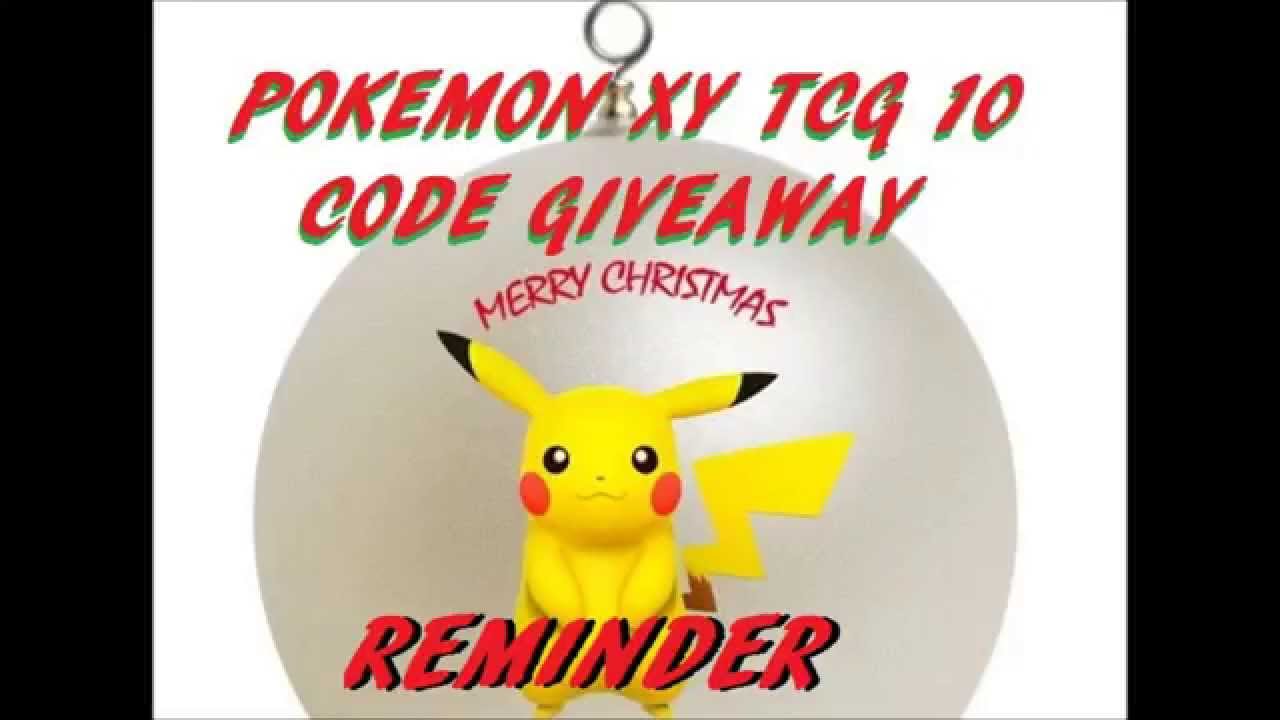In this image, an advertisement for a giveaway is prominently displayed. The text is written in bold red font on a predominantly white background, announcing a "Pokemon XY TCG 10 Code Giveaway." At the center of the image is a silver, round bulb-style Christmas tree ornament, featuring an illustration of the Pokémon character Pikachu. Above Pikachu's head, in delicate red lettering, are the words "Merry Christmas." The ornament and overlay text are set against the simple, clean white background, highlighting the festive theme and the specifics of the giveaway. A reminder about the giveaway is included at the bottom of the image, reinforcing the promotional message.